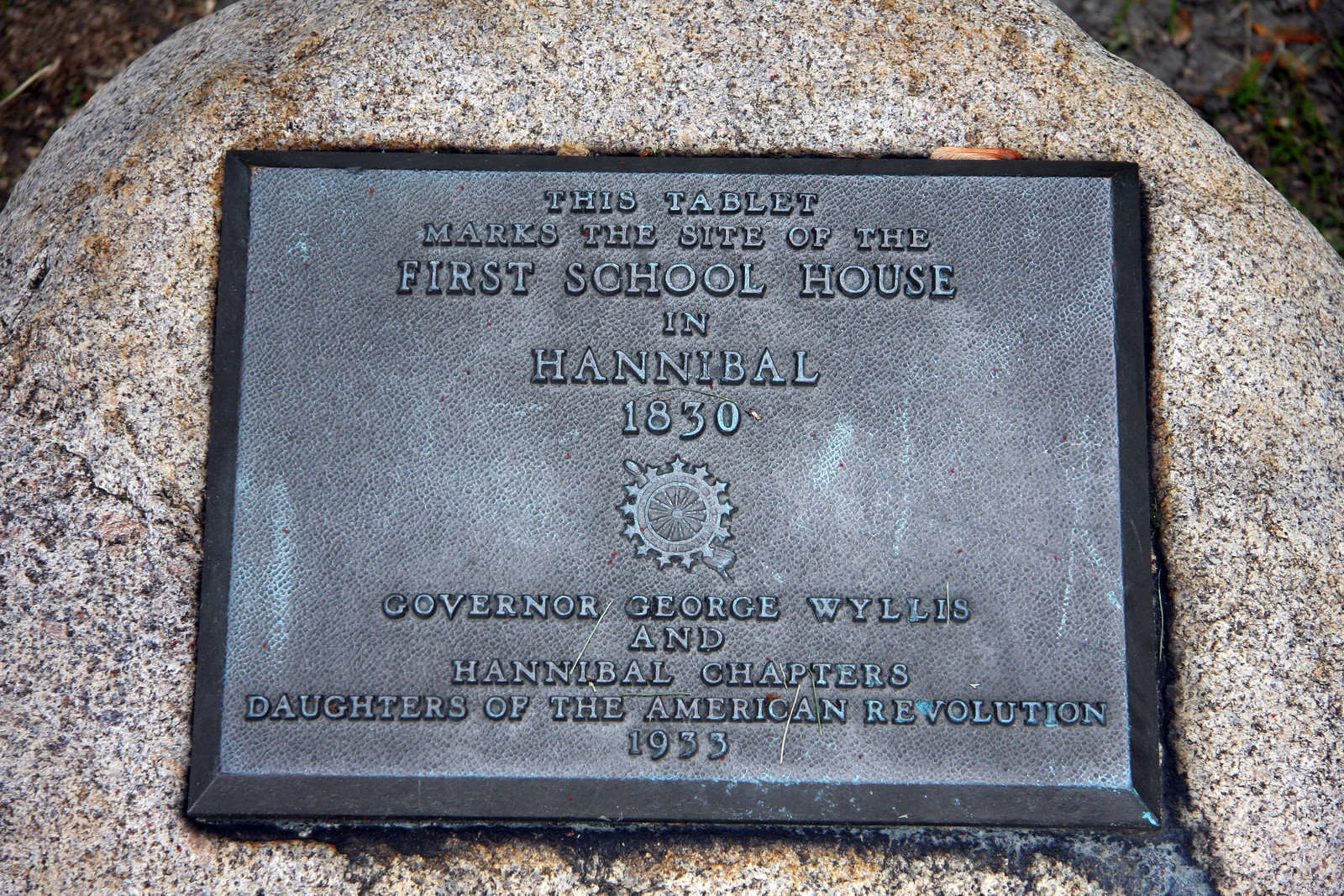The image captures a historical marker that commemorates the first schoolhouse in Hannibal from the year 1830. The marker is a rectangular metal plaque, featuring raised lettering and affixed to a large spherical rock set against a bare, dark brown dirt ground. The plaque, light gray with dark gray outlining, bears the inscription: "This tablet marks the site of the first schoolhouse in Hannibal, 1830." Below this text, a stylized ship's steering wheel symbol is depicted, followed by the additional inscription: "Governor George Willis and Hannibal Chapters, Daughters of the American Revolution, 1933." Several black trail marks are evident at the junction where the plaque meets the rock.